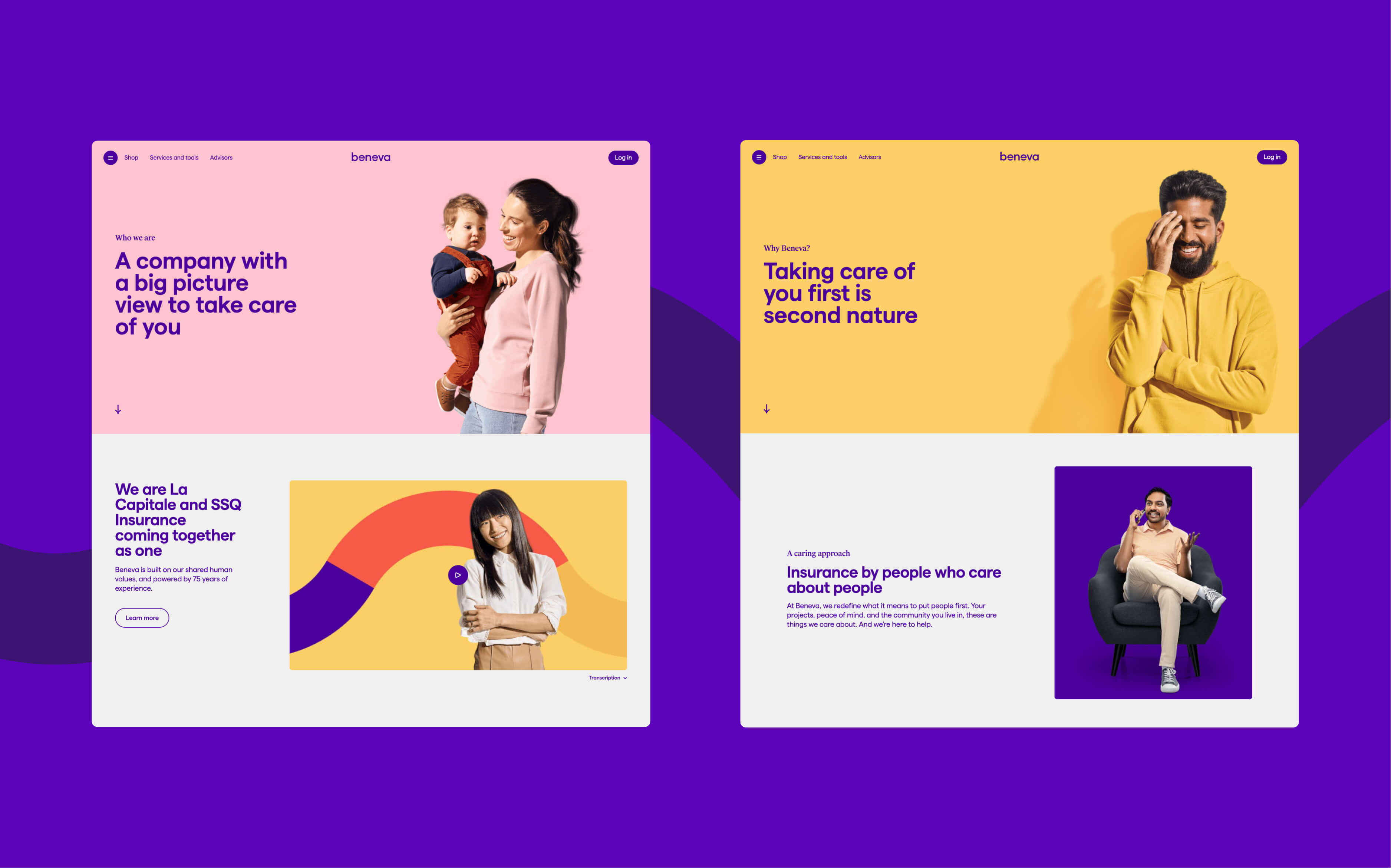**Caption:**

The image features a detailed composite of two advertisements placed side by side for Beneva, an insurance company. Each section encompasses distinct visual and textual elements aimed at conveying the brand's message and services.

**Left Advertisement:**
- **Background Colors:** The upper and lower sections are set against pink and white backgrounds respectively.
- **Textual Elements:** 
  - The top left corner includes a blue circle with a hamburger menu icon.
  - Next to it, the words "Shop Service and Tools Advisors" are prominently displayed.
  - To the right, the word "Log In" is visible.
  - The brand name "Beneva" is centered.
  - Underneath, larger text reads "Who We Are," followed by the phrase "Acccompany *a big-picture view to take care of you*", adding a rhyming touch.
- **Visual Elements:**
  - At the center is a heartwarming photograph of a woman and a baby:
    - The baby is dressed in brown coveralls, a long-sleeved blue shirt, and brown shoes.
    - The woman, possibly the baby's mother, has long brown hair tied back in a ponytail and is wearing a pastel pink sweater and blue jeans. She holds the baby with her right hand and smiles at him.
- **Bottom Section:**
  - The image of another woman, who appears to be of Asian descent, with long black hair, is displayed against a yellow background.
  - She is dressed in a white blouse and brown slacks.
  - Left-aligned text reads: 
    - "We Are La Capital and SSQ Insurance, coming together as one. Beneva is built on our shared human values and powered by 75 years of experience."
    - Below, there is a clickable oval button that says "Learn More.”

**Right Advertisement:**
- **Background Colors:** Features a harmonious blend of yellow and white backgrounds.
- **Textual Elements:**
  - The upper section again includes "Shop Service and Tools Advisors," the brand name "Beneva," and the "Log In" text.
  - The phrase "Why Beneva?" and the sentiment "Taking care of you first is second nature" emphasize the company's customer-focused approach.
- **Visual Elements:**
  - Top photograph showcases a man with medium-dark brown skin, laughing. 
    - He is wearing a yellow hoodie, and his short, wavy dark hair is complemented by a well-trimmed mustache and beard. 
    - His right hand covers his eye as he laughs heartily.
  - Bottom section text reads "A Caring Approach. Insurance by people who care about people. At Beneva, we redefine what it means to put people first. Your projects, peace of mind, and the community you live in. These are things we care about, and we're here to help."
  - Adjacent visual portrays a man sitting in a soft, cushiony gray armchair with black legs.
    - He is dressed in light-colored pants and a pastel pink short-sleeved shirt.
    - Holding a cell phone to his ear with his right hand, he gestures with his left hand, suggesting active conversation or engagement.

Overall, this advertisement underscores Beneva's commitment to customer care and human-centric values through a confluence of engaging visuals and thoughtful text.